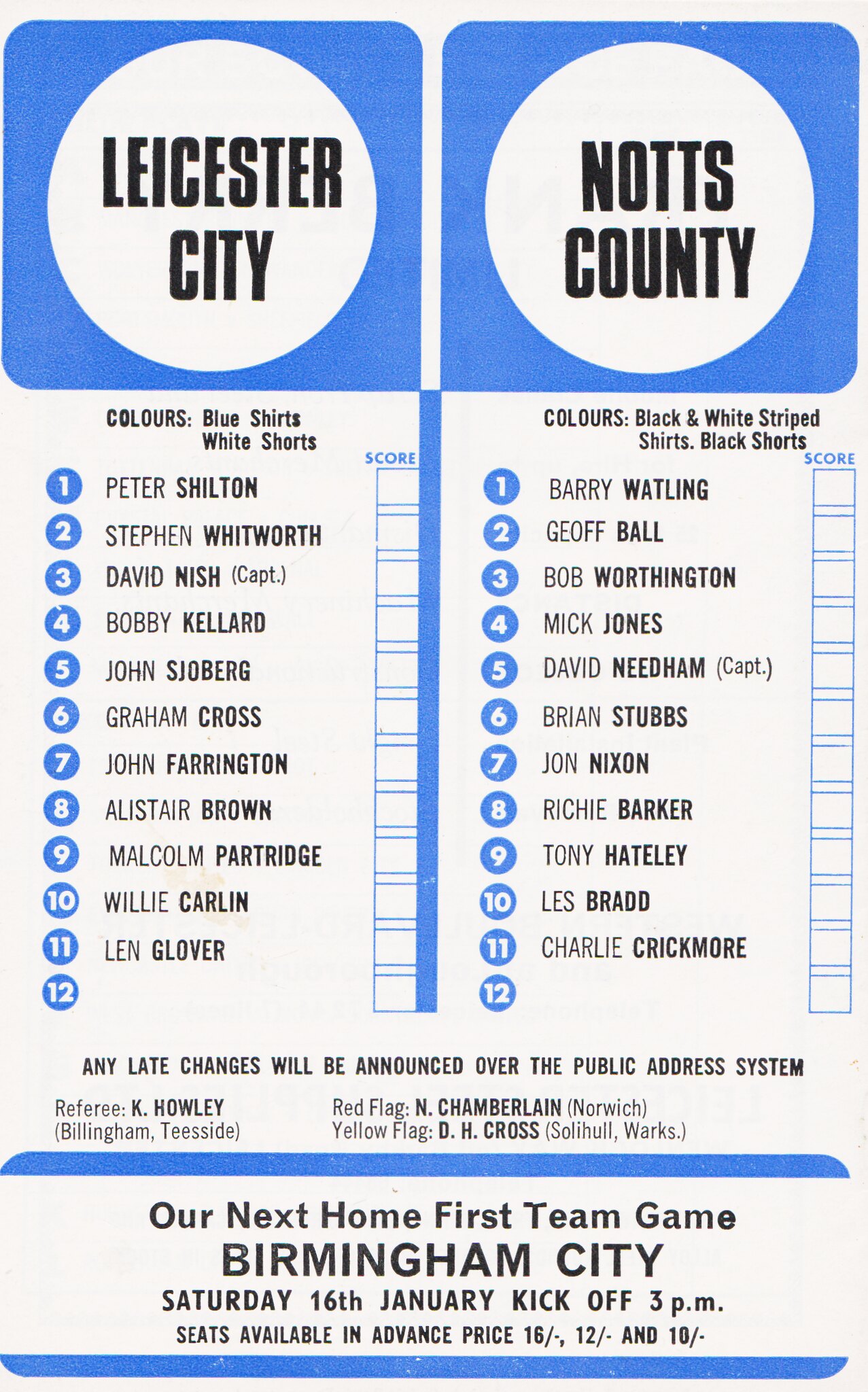The image is an advertisement for an upcoming event featuring a detailed match program for two football teams: Leicester City and Knott's County. The layout features two columns of information, each dedicated to one team. At the top of the image are two blue squares, each enclosing a white circle with black text. The left square reads "Leicester City" and the right one reads "Knott's County."

Directly below, the team colors are listed: Leicester City wears blue shirts and white shorts, while Knott's County wears black and white striped shirts with black shorts. 

Following this, the player line-ups for each team are presented. For Leicester City:
1. Peter Shilton
2. Stephen Whitworth
3. David Nish (captain)
4. Bobby Kellard
5. John Sjoberg
6. Graham Cross
7. John Farrington
8. Alistair Brown
9. Malcolm Partridge
10. Willie Carlin
11. Len Glover
12. (No name)

For Knott's County:
1. Barry Watling
2. Geoff Ball
3. Bob Worthington
4. Mick Jones
5. David Needham (captain)
6. Brian Stubbs
7. John Nixon
8. Richie Barker
9. Tony Hateley
10. Les Bradd
11. Charlie Crickmore

Below the player lists, the text indicates: "Any late changes will be announced over the public address system." It also provides details about the officials for the game: the referee is K. Howley from Billingham, Teesside; the red flag official is North Chamberlain from Norwich; and the yellow flag official is D.H. Cross from Solihull Works.

At the bottom of the image, within a rounded rectangle with a blue outline, is an announcement for the next home first team game: "Birmingham City, Saturday, 16th January, kickoff 3 p.m. Seats available in advance, price 16/12 and 10/nothing."